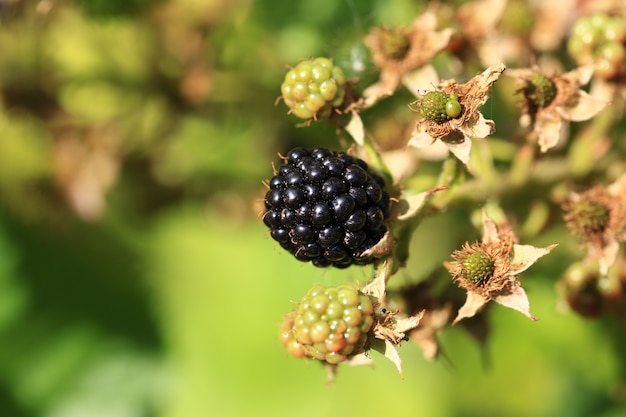In this detailed close-up image of a blackberry bush, taken outdoors in the daytime, the focus rests on a single ripe blackberry at the center. This fully grown, dark-hued berry is flanked by various stages of unripe berries. To the right of the ripe blackberry, clusters of smaller green berries are visible, gradually maturing but not yet ready to be picked. Below the central berry, another green berry, which is about half the size, can be seen. Surrounding these are buds and straw-like brown elements. The background features a blend of blurred bright green and dark gray colors, adding a natural, soft-focus effect to the setting. There is no text in the image, and the sharp focus on the ripe blackberry contrasts with the slightly out-of-focus unripe berries and foliage, capturing the essence of a vibrant nature setting.